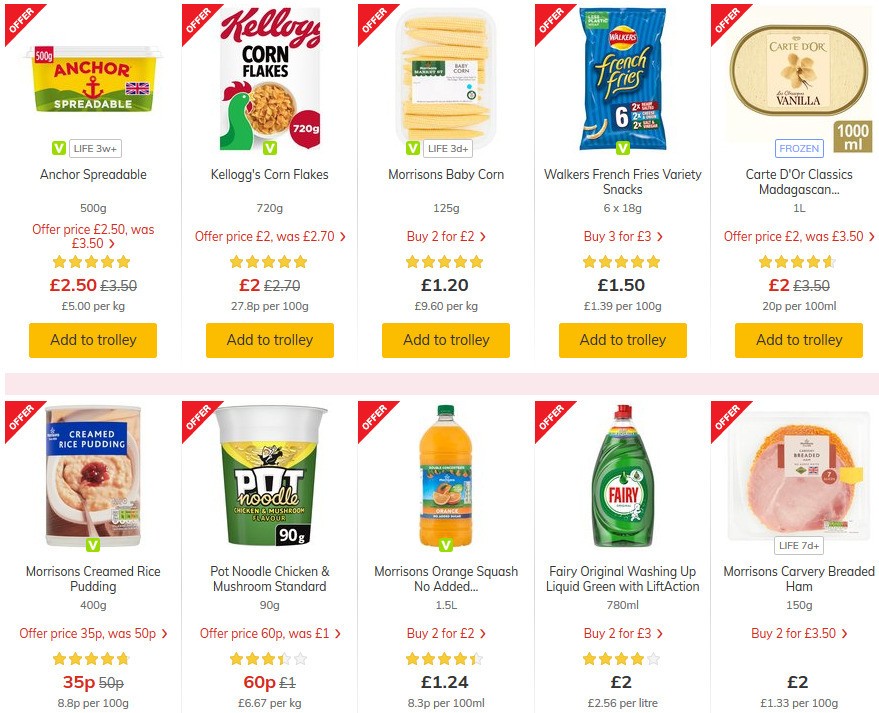This image is a detailed screenshot from a Morrison's supermarket website, showcasing a variety of products with special offers. The background is primarily white, with a red triangle featuring the word "OFFER" in white capital letters at a slanted angle on the top corner of each product image.

**Top Row (Left to Right):**
1. **Anchor Spreadable Butter Tub**
   - **Annotation:** Life 3 Weeks Plus
   - **Weight:** 500g
   - **Offer Price:** £2.50 (previously £3.50, in grey with a strike-through)
   - **Unit Price:** £5 per kilo
   - **Rating:** 5 gold stars
   - **Add to Trolley:** Yellow button with black text

2. **Kellogg's Corn Flakes**
   - **Weight:** 720g
   - **Offer Price:** £2.00 (previously £2.70, in grey with a strike-through)
   - **Unit Price:** 27.8p per 100g
   - **Rating:** 5 gold stars
   - **Add to Trolley:** Yellow button with grey text

3. **Morrison's Baby Corn**
   - **Weight:** 125g
   - **Offer Detail:** Buy 2 for £2
   - **Price:** £1.20
   - **Unit Price:** £9.60 per kilo
   - **Rating:** 5 gold stars
   - **Add to Trolley:** Yellow button with grey text

4. **Walker's French Fries Variety Snacks**
   - **Pack Size:** 6 x 18g
   - **Offer Detail:** Buy 3 for £3
   - **Price:** £1.50
   - **Unit Price:** £1.39 per 100g
   - **Rating:** 5 gold stars
   - **Add to Trolley:** Yellow button with grey text

5. **Carte D'Or Vanilla Ice Cream**
   - **Annotation:** Frozen
   - **Volume:** 1L
   - **Full Name:** Carte D'Or Classics Madagascan Vanilla
   - **Offer Price:** £2.00 (previously £3.50, in grey with a strike-through)
   - **Unit Price:** 20p per 100ml
   - **Rating:** 4.5 gold stars
   - **Add to Trolley:** Yellow button with grey text

**Bottom Row (Left to Right):**
1. **Morrison's Cream Rice Pudding**
   - **Weight:** 400g
   - **Offer Price:** 35p (previously 50p, in grey with a strike-through)
   - **Unit Price:** 8.8p per 100g
   - **Rating:** 4.8 gold stars
   - **Add to Trolley:** Yellow button with grey text

2. **Pot Noodle - Chicken and Mushroom**
   - **Weight:** 90g
   - **Offer Price:** 60p (previously £1.00, in grey with a strike-through)
   - **Unit Price:** £6.67 per kilo
   - **Rating:** 3.25 gold stars
   - **Add to Trolley:** Yellow button with grey text

3. **Morrison's Orange Squash**
   - **Volume:** 1.5L
   - **Offer Detail:** Buy 2 for £2
   - **Price:** £1.24
   - **Unit Price:** 8.3p per 100ml
   - **Rating:** 4.25 gold stars
   - **Add to Trolley:** Yellow button with grey text

4. **Fairy Original Washing Up Liquid**
   - **Volume:** 780ml
   - **Offer Detail:** Buy 2 for £3
   - **Price:** £2.00
   - **Unit Price:** £2.56 per litre
   - **Rating:** 4 gold stars
   - **Add to Trolley:** Yellow button with grey text

5. **Morrison's Carvery Breaded Ham**
   - **Annotation:** Life 7 Day Plus
   - **Weight:** 150g
   - **Offer Detail:** Buy 2 for £3.50
   - **Price:** £2.00
   - **Unit Price:** £1.33 per 100g
   - **Add to Trolley:** Yellow button with grey text

This detailed display allows customers to easily discern the offers, product details, and prices, encouraging informed purchasing decisions.